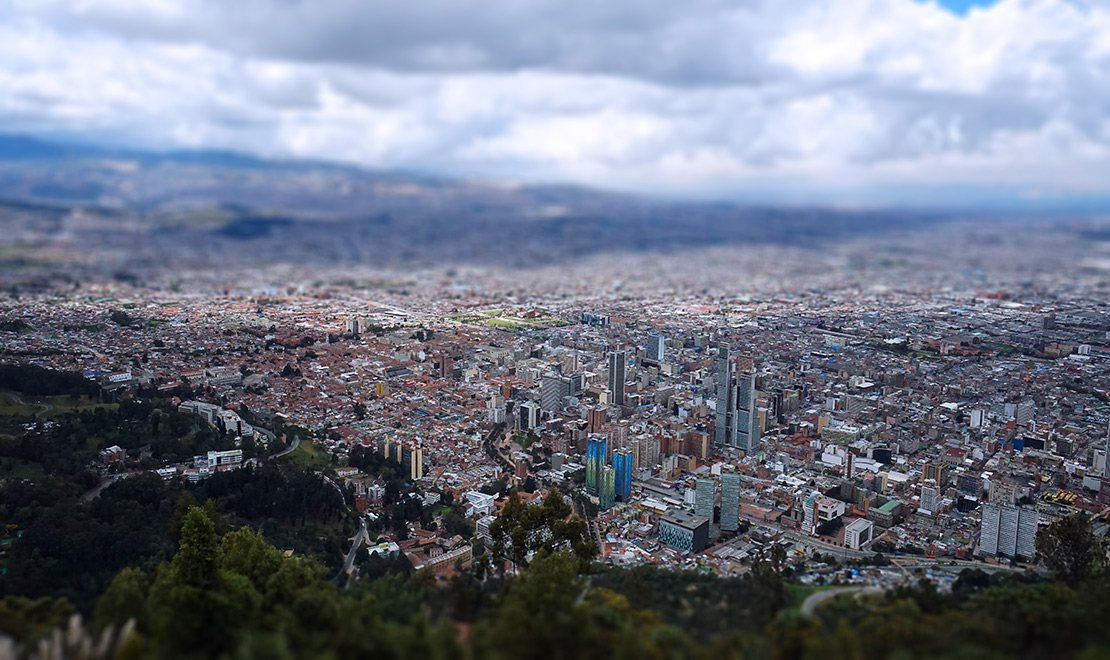The photograph captures a vast, sprawling cityscape extending all the way to the horizon, taken from a vantage point high on a hill. The densely populated urban area is blanketed with buildings of various sizes, from towering skyscrapers concentrated in the center to shorter structures as one moves outward. Many of the buildings feature white siding and roofs of reddish clay hues, interspersed with striking blue high-rises. The bottom left corner and lower edge of the image reveal lush green vegetation, including trees and shrubs, marking the hill from which the city is viewed. The sky above, mostly covered with thick, white clouds with dark undersides, allows glimpses of blue. Far in the distance, on the top left, the contours of mountains frame the city, which stretches to their foothills, emphasizing the immense size and density of the urban sprawl.